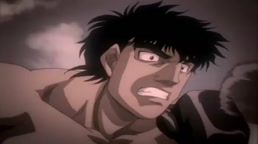This image shows a detailed cartoon drawing of a man, positioned in a small rectangular frame. The man's head is prominently featured in the center of the image, facing forward and slightly to the right. His medium-length black hair is messy and spiky, jutting out in various directions. His intense, wide-open eyes, which appear white with black pin-drop pupils, and thick black eyebrows contribute to his visibly angry expression. His mouth is open, revealing a grimace with clenched teeth. The man's neck and part of his upper body are visible below his head, with his body extending off the page to the bottom middle and middle left. The background depicts a gray sky with white clouds to his left. To the right of the man, there is a gray box-like object, possibly part of his surroundings, and something that might be a tree entering from the right edge of the frame. The overall color scheme includes dark, two-tone browns, tans, and light highlights, giving the image a dramatic and intense atmosphere.